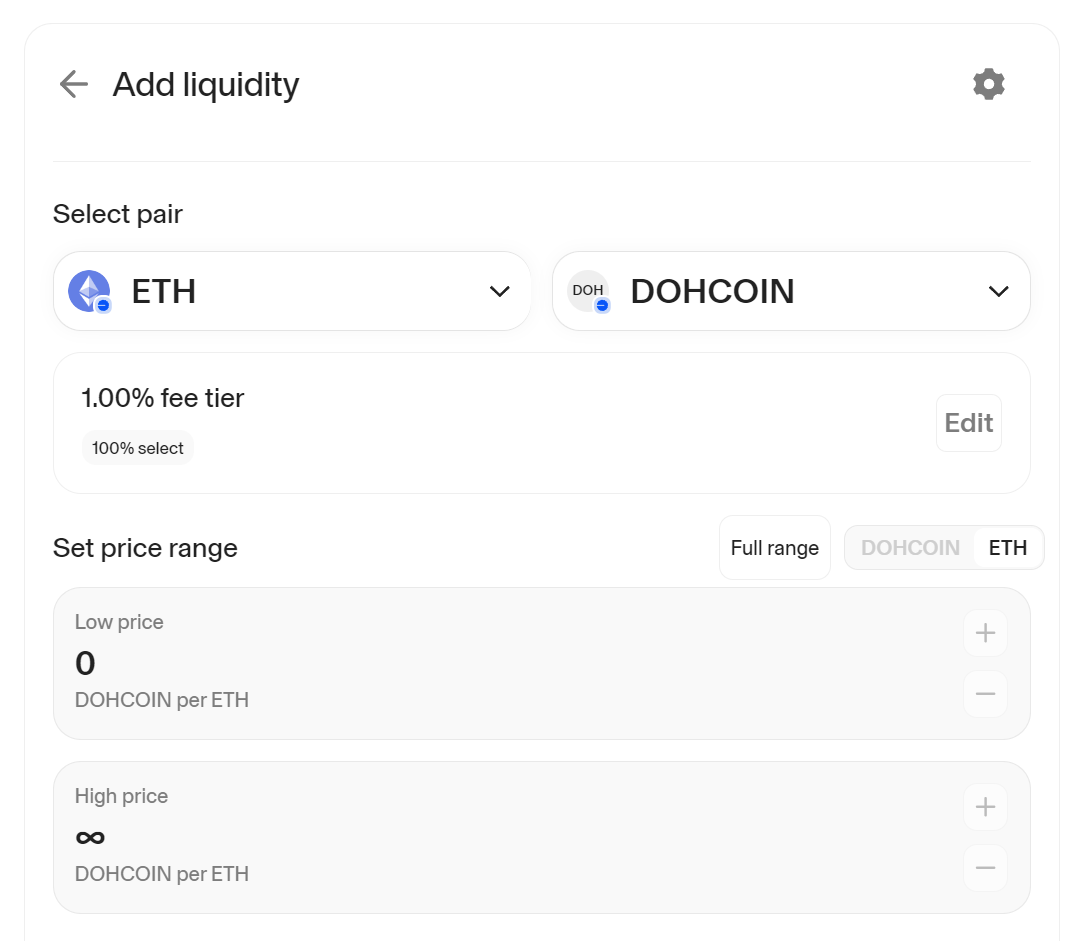The image depicts a user interface of a cryptocurrency platform focused on adding liquidity. The background is a white webpage. At the top, the heading "Add Liquidity" is prominently displayed. To the left of the heading, there is a gray arrow icon, and to the right, a gray settings wheel icon.

Below the heading, the text "Select Pair" is written in black. Beneath this, there are two dropdown menus. The first dropdown is for selecting 'ETH' (Ethereum), accompanied by its purple and white diamond-like logo with a blue circle at the bottom. The second dropdown is for selecting 'DOH Coin,' which is represented by its own circular logo with a blue circle at the bottom.

The interface shows a fee tier set at 1% and indicates that 100% has been selected. There is an edit button available for this section. Following this, the text "Select Price Range" appears in black, alongside an option labeled "Full Range" to the right.

Further details include blurred representations of DOH Coin and ETH in the price range settings. The "Set Price Range" section shows a low price point at 0 DOH coin per ETH, with plus and minus buttons for adjusting the values, and a high price point remaining unspecified.

Overall, the interface provides tools for users to configure various settings related to adding liquidity in a cryptocurrency context.